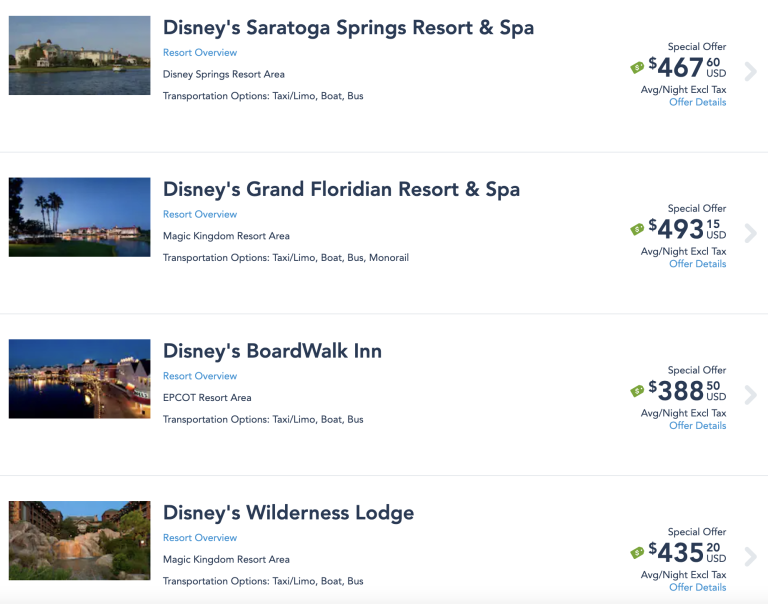The screenshot showcases a website featuring four different hotel listings, all associated with Disney. Each listing is organized with a prominent image, hotel name, resort overview link, location within Disney, transportation options, and special pricing details.

1. **Disney's Saratoga Springs Resort & Spa**
   - **Image:** Scenic view likely of a lake or ocean.
   - **Resort Overview:** Linked text.
   - **Location:** Disney Springs Resort Area.
   - **Transportation Options:** Taxi/Limo, Boat, Bus.
   - **Special Offer:** $467.60 USD per night (average, excluding tax). An "Offer Details" link and a gray arrow for more information.

2. **Disney's Grand Floridian Resort & Spa**
   - **Image:** Palm trees creating a tropical ambiance.
   - **Resort Overview:** Linked text.
   - **Location:** Magic Kingdom Resort Area.
   - **Transportation Options:** Taxi/Limo, Boat, Bus, Monorail.
   - **Special Offer:** $493.15 USD per night (average, excluding tax).

3. **Disney's BoardWalk Inn**
   - **Image:** Not specified in detail.
   - **Resort Overview:** Linked text.
   - **Location:** Epcot Resort Area.
   - **Transportation Options:** Taxi/Limo, Boat, Bus.
   - **Special Offer:** $388.50 USD per night (average, excluding tax).

4. **Disney's Wilderness Lodge**
   - **Image:** Not specified in detail.
   - **Resort Overview:** Linked text.
   - **Location:** Magic Kingdom Resort Area.
   - **Transportation Options:** Taxi/Limo, Boat, Bus.
   - **Special Offer:** $435.20 USD per night (average, excluding tax).